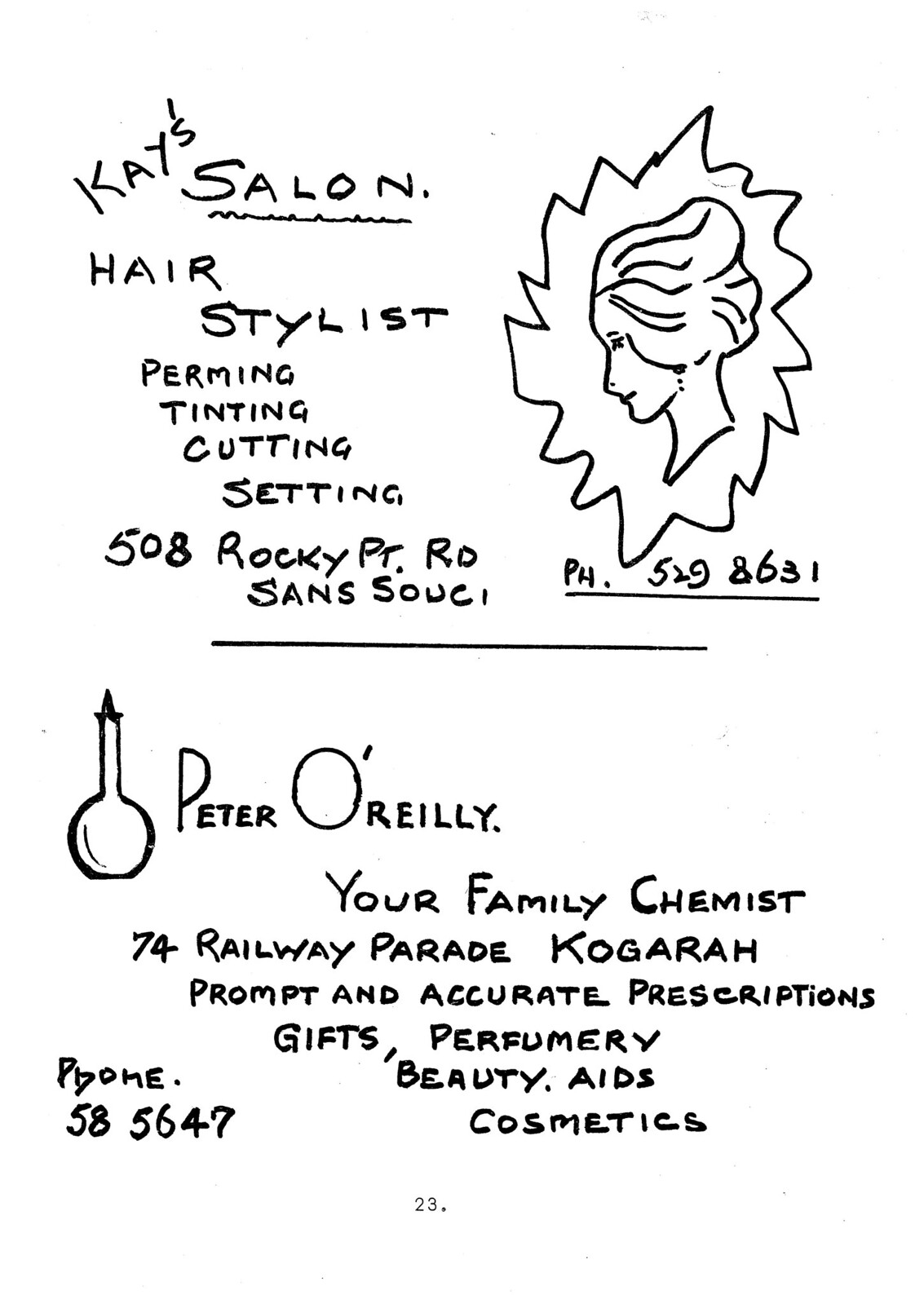The hand-drawn image features two distinct advertisements on a white background with black text. The top advertisement, positioned in the upper part of the image, promotes "K's Salon" with the name written diagonally from left to right and underlined with a jagged line. Below the salon's name, the text "Hairstylist, Perming, Tinting, Cutting, Setting" is written diagonally with each service starting a new line. The address "508 Rocky Point Road, Sansui" and a phone number "549-8631" (although there is some discrepancy in the digits) are included. Accompanying the text is a hand-drawn illustration of a cartoon girl or mannequin head with a fancy, fluffy hairdo, pointed to the left and outlined with a leafy texture.

The lower advertisement is for "Peter O'Reilly, Your Family Chemist" located at "74 Railway Parade, Kogara (alternatively mentioned as Cougar Rock or Kogara)," featuring services such as prompt and accurate prescriptions, gifts, perfumery, beauty aids, and cosmetics. The phone number for Peter O'Reilly's chemist is listed as "58 5647" (with minor variations mentioned). Both advertisements are neatly stacked and well-spaced, making the text easy to read, all set in a hand-drawn style that gives a cohesive and artistic feel to the overall design.